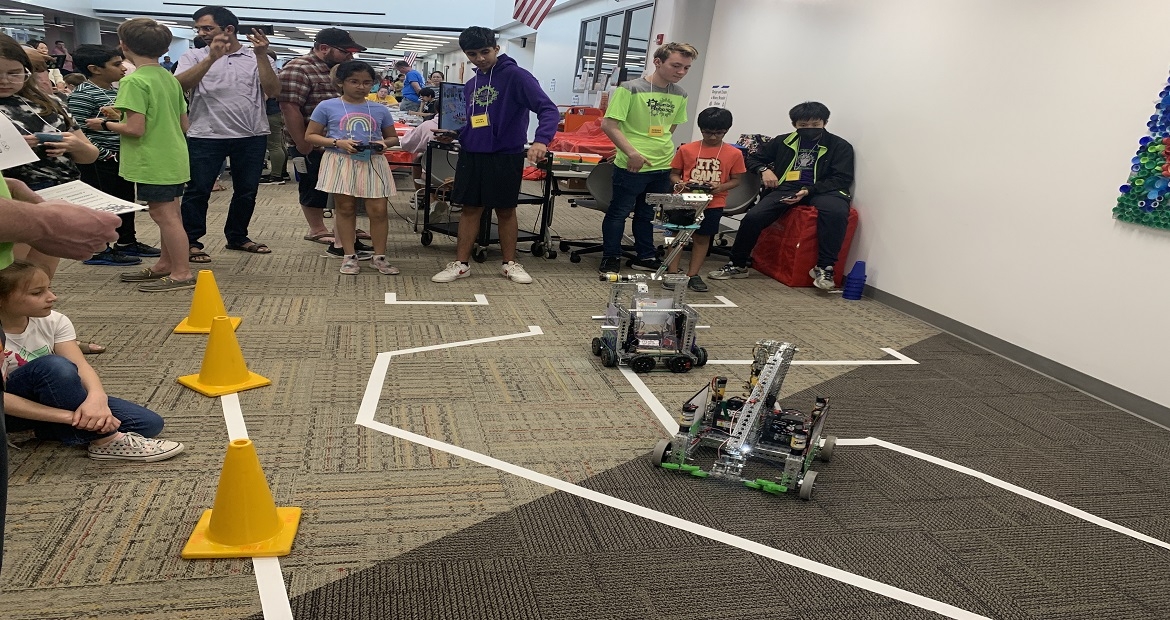In a bustling convention center corridor, a group of children and a few adults are immersed in a robotics competition. The photograph captures a vibrant scene with a mix of boys and girls, predominantly aged 10 to 13, scattered around a makeshift obstacle course marked with white tape on a transitioning gray-to-tan carpet. At the center of activity, two kids, one with black hair donning an orange shirt emblazoned with "It's Game," maneuver their remote-controlled robots — one a box-like vehicle with a prominent metal bar designed for smashing, the other an open box structure missing two walls, with a slide-like bar inside. Spectators, some with handheld controllers, gather around the taped-off arena bordered by three yellow cones. An adult in a facemask animatedly gestures, possibly giving instructions or guidance, while another, potentially a judge, equipped with glasses and a phone, observes the action from the top left corner. The atmosphere echoes the excitement of a BattleBots episode, amplified by the involvement and curiosity of the surrounding crowd.